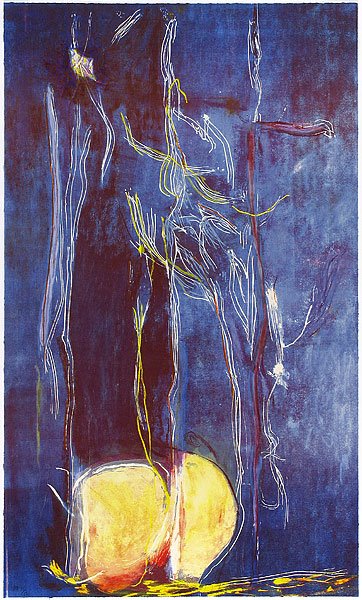This image showcases a highly abstract piece of art dominated by a cobalt blue background, accented with a darker blue stripe that stretches vertically about three-quarters to the left. Towards the bottom, a vibrant yellow line is scratched across the canvas, accompanied by two yellow half-circles just above it, which somewhat resemble a pair of buttocks merging with the dark blue stripe. Throughout the artwork, white and red lines are etched sporadically from top to bottom, contributing to the chaotic yet deliberate design. The color palette extends to include light blue, purple, orange, black, and white, though these hues are less prominent. The painting lacks any identifiable objects, text, or scenery, embodying a random, imaginative style that feels reminiscent of youthful, uninhibited creativity.